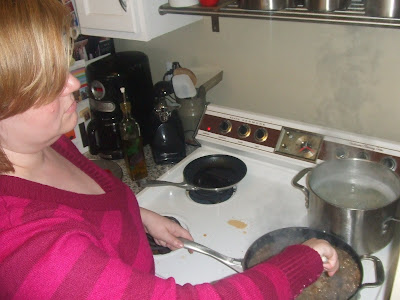A woman with reddish-brown hair, parted to the side and cut to just below her ears, is intently cooking at an old-fashioned white stove. Wearing a long-sleeve sweater adorned with horizontal light and dark purple stripes, she uses her left hand to steady a frying pan while her right hand stirs what appears to be ground beef. Behind her frying pan, a pot of water boils away, and an empty frying pan sits idle on the stove's back left burner. The stove features wood grain around the knobs, hinting at its aged design. To the left of the stove is a countertop housing a coffee maker, a bottle of olive oil, and a few ceramic containers. Above the stove, a spice rack adds a touch of organization, and a white cabinet door is slightly ajar, revealing more storage space. The scene captures a moment of focused culinary activity in a cozy kitchen setting.